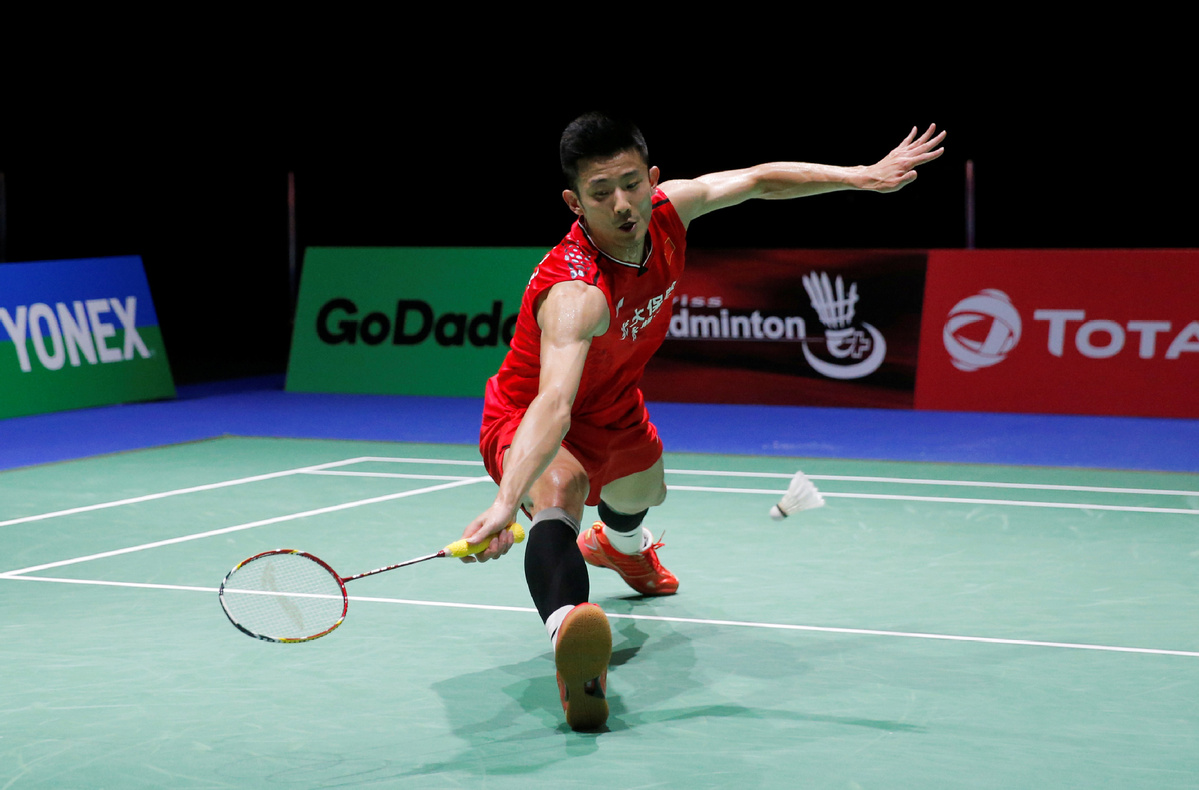In this photograph, an Asian man is captured mid-action on a green badminton court marked with white lines. He is intensely focused as he leans to his right with his right leg extended, the heel touching the ground, getting ready to hit a white shuttlecock with his yellow-handled racquet. The player is donned in a red and white jersey with red shorts, complemented by black socks and orange-red shoes. The backdrop features various boundary boards, including ones with the texts "YONEX," "Go Daddy," and "TOT" emblazoned in white letters on red backgrounds, along with a symbolic shuttlecock and some additional signage. In the far background, two vertical objects reflecting light are visible against the otherwise dark setting. The scene is singularly focused on the player, emphasizing his athletic poise and concentration in the sport.